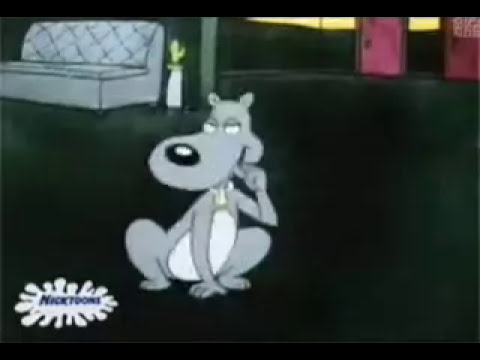The image features a detailed cartoon scene centered around a stylized dog with a gray body, white belly, and black nose. The dog, which has heavy-lidded eyes and a prominent snout that appears larger than its body, is positioned slightly off-center to the left, squatting on a dark, greenish-black floor. Behind the dog, in the top-left corner, is a gray couch, with a pot holding a lime-green plant positioned just below it. In the background, there are two pink doors located in the top-right corner, one slightly to the left of the other, with a hint of light suggesting windows above them. The bottom left of the image features a Nicktoons logo in black and white. The scene is framed by thin black borders at the top and bottom, contributing to the overall cartoon aesthetic.